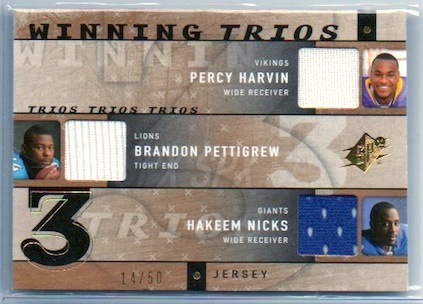The image is a detailed color photograph of a packaged product featuring three NFL players, labeled as "Winning Trios." The packaging appears to be around 3 inches tall and 5 inches wide, covered in transparent wrapping. The top part of the package prominently features the title "Winning Trios" in black capitalized letters. Below this title, the image is divided into three sections, each showcasing a different player from a different NFL team.

The top section highlights Percy Harvin, a wide receiver from the Minnesota Vikings, depicted smiling in his Vikings t-shirt. Next to his image, there's a small window displaying a white item, possibly sticky tape.

The middle section features Brandon Pettigrew, a tight end from the Detroit Lions, wearing his blue Lions uniform. Beside his image, there is another window showing a white square with vertical indentations, probably indicating another type of material.

The bottom section displays Hakeem Nicks, a wide receiver from the New York Giants, also in his blue uniform. To the left of his photo is a blue square with lighter blue dots.

Each section includes a large stylized number three in various positions, integrated into the background design, which features the word "TRIOS" in large pale letters. At the bottom of the image, the text reads "14/50 JERSEY," indicating that this is the 14th item out of a 50-item limited edition. Brandon Pettigrew is also seen holding a football, adding a dynamic element to the composition.

The background behind the athletes features elements that resemble a large stylized number three, tying in with the theme of trios. The inclusion of different textures and materials in small windows next to each player suggests that the product may be showcasing samples or parts of jerseys associated with these players. The players' darker skin tones are noticeable, confirming that all three athletes are African-American.